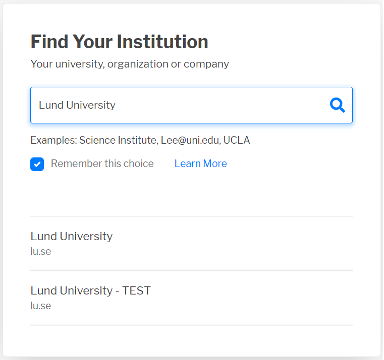This image features a white screen bordered by a thin gray line. Positioned just below the top border on the upper left-hand side, the bold black text reads "Find Your Institution" with capitalized initials: F, Y, and I. Beneath this, in smaller font, it prompts users to "Enter your university, organization, or company." Further down, a search bar displays "London University" left-aligned within the bar, accompanied by a blue magnifying glass icon on the right side of the search bar.

Following the search bar, a checkbox is marked beside the text "Remember this choice". Below this checkbox, an option to "Learn more" is presented in blue text. Further down, "London University" is displayed prominently, with the associated website "lu.se" in smaller font underneath. Finally, the term "London University - Test" appears at the bottom of the screen in smaller text.